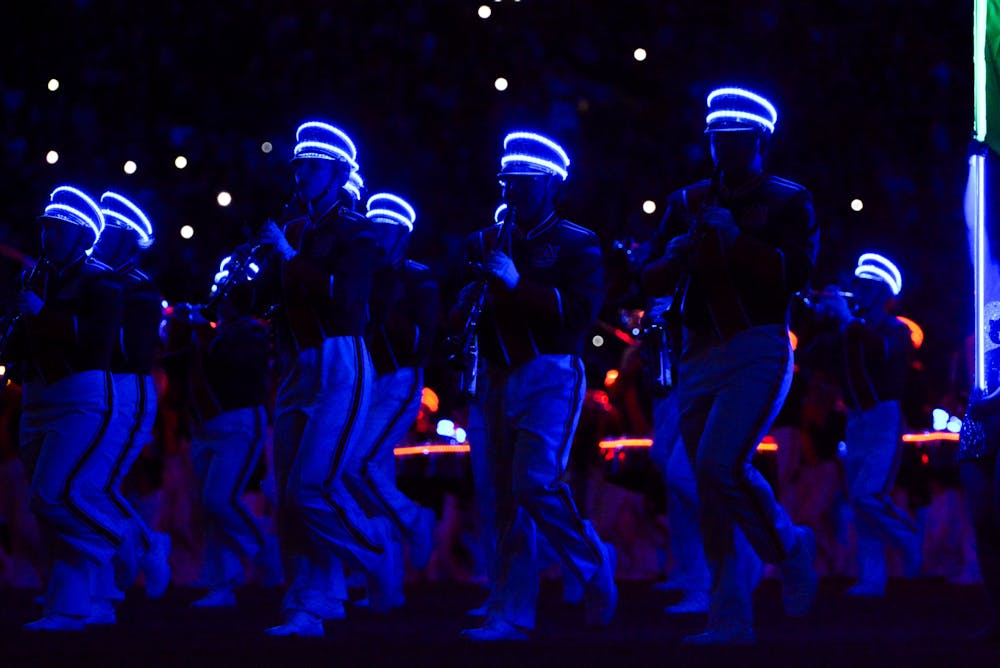This image captures a vibrant marching band, illuminated by a striking interplay of neon lights against a dark backdrop. The band members are all dressed in predominantly white uniforms accented by blue stripes on their pants. Their distinct headgear features neon lights in blue and purple hues, encircling the caps and creating a visually captivating effect. Each musician, mostly playing clarinets and horns, contributes to the dynamic scene as they march from right to left. In the background, a mixture of neon lights in orange, purple, and green enhances the atmospheric depth. The overall color theme of the image is dominated by blue and white, with additional lighting effects adding a spectrum of colors, providing a vivid and electric ambiance.